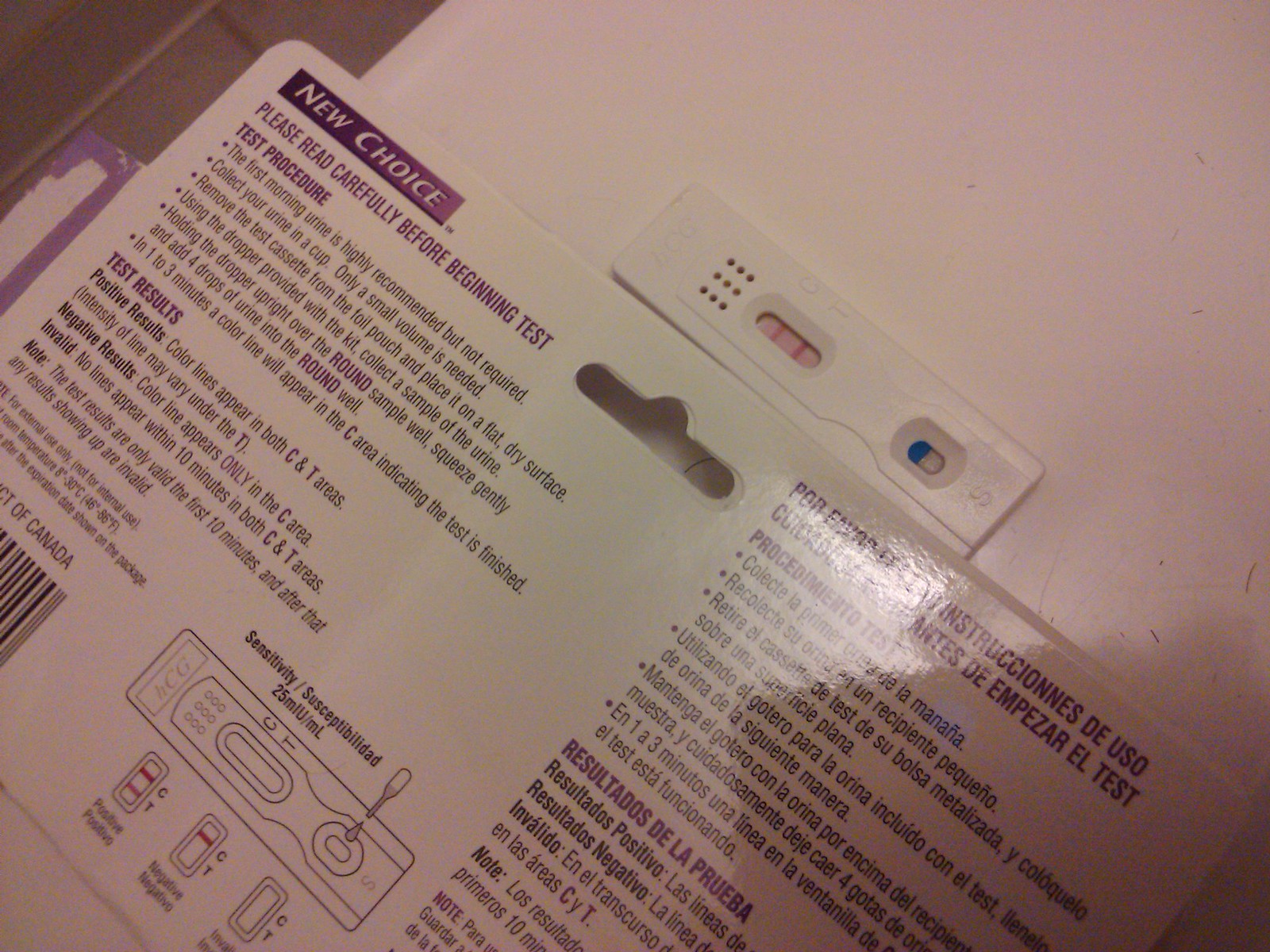This is an image of an individual administering what appears to be a pregnancy test. Upon closer inspection of the box labeled "New Choice," it becomes clear that this is indeed a pregnancy test kit. The detailed instructions on the box advise users to read carefully before starting the test. It is recommended, although not required, to use the first morning urine for optimal results. The procedure involves collecting a small sample of urine in a cup and then using the provided dropper to add four drops into the sample well on a flat, dry surface.

The instructions indicate that within one to three minutes, a color line will appear in the C (control) area, signaling the test is complete. Test results are interpreted as follows: 
- Positive: Color lines appear in both the C and T (test) areas, with the intensity of the T line possibly varying. The test in the image shows a much stronger T line, indicating a positive pregnancy result.
- Negative: A color line appears only in the C area.
- Invalid: No lines appear in either the C or T areas within 10 minutes.

The image also shows the test cassette on the right-hand side with a visible thicker line for the T area and a line for the C area, and an additional blue area labeled S. Notably, the instructions on the box are also provided in Spanish on the right-hand side.